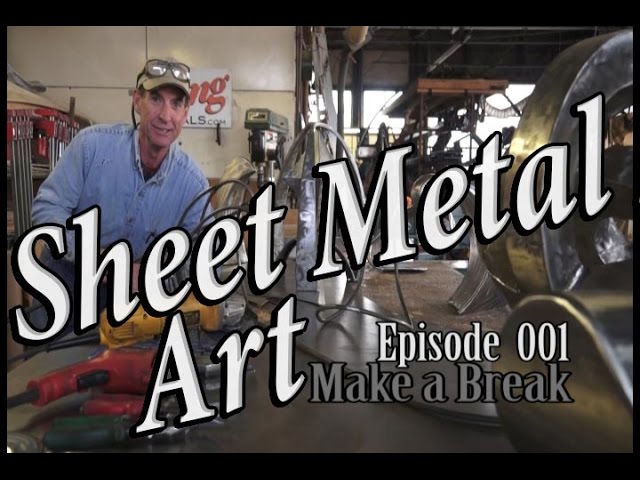The image is a detailed screenshot from the opening screen of a YouTube video titled "Sheet Metal Art, Episode 001: Make a Break." The large white text overlays the scene, clearly marking it as a promotional still for the video. The background reveals a metalworking shop, filled with heavy machinery used for bending and breaking sheet metal. Centered in the scene, a man resembling Bill Nye the Science Guy is smiling while leaning over a table cluttered with large pieces of metal and various power tools. He is wearing a tan-colored baseball cap with safety goggles perched atop, and a button-up denim long-sleeve shirt. On the table in front of him, there are two electric grinders, one yellow and one red. The overall setting emphasizes a professional and industrious environment dedicated to metalworking craft.